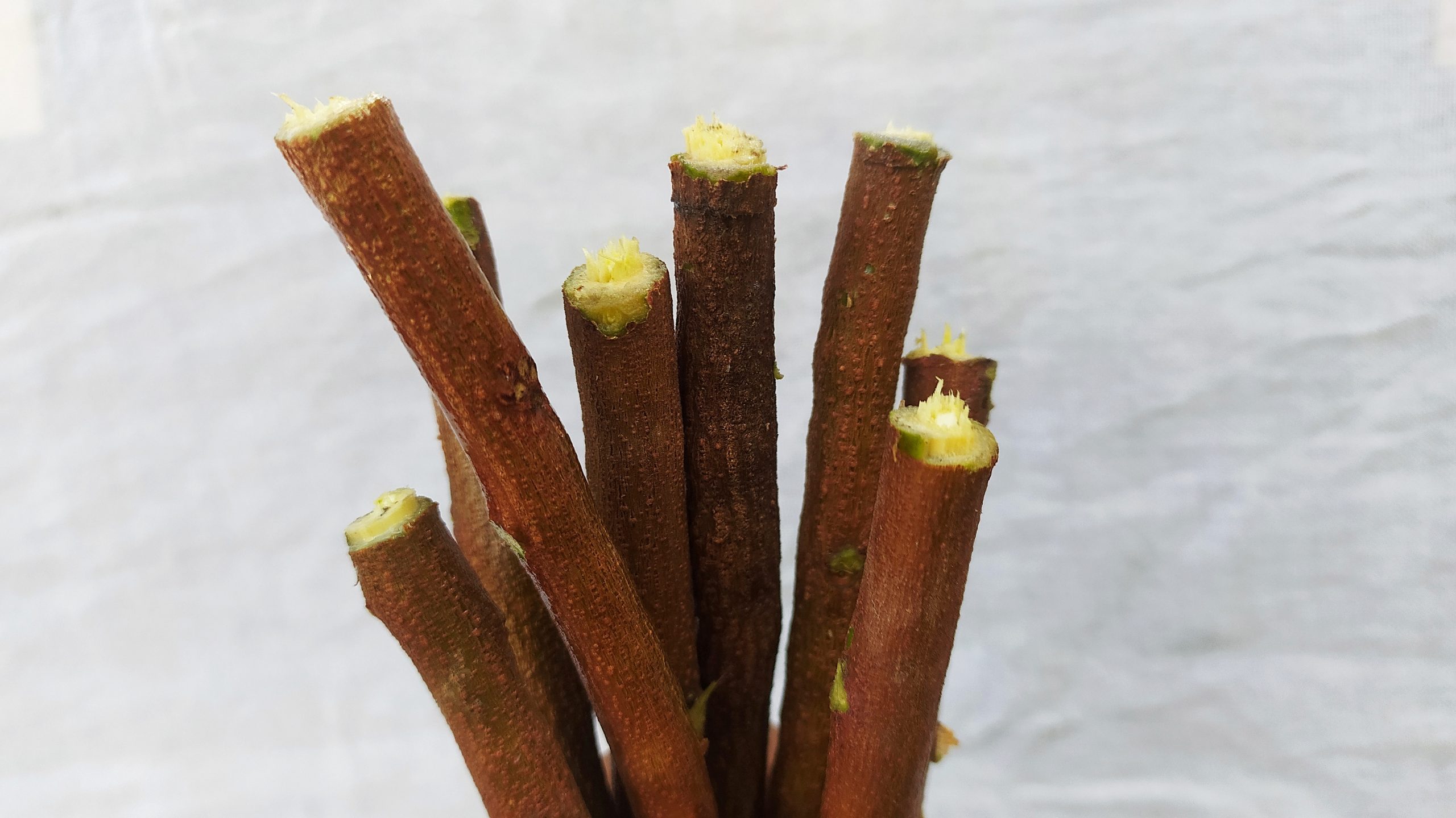This image features a close-up of eight roughly cut brown sticks or branches, varying in length. The cut ends reveal a fibrous core, appearing damp and displaying hues of tan, yellow-green, and reddish tones. Some of the branches have smaller offshoots that were also trimmed. The background resembles a crinkled white or gray cloth, giving the impression of an uneven surface similar to an unironed sheet. The fibrous interior of the branches has a slightly spiky texture, which might indicate recent water exposure, similar to the wet look of freshly cut pineapple.